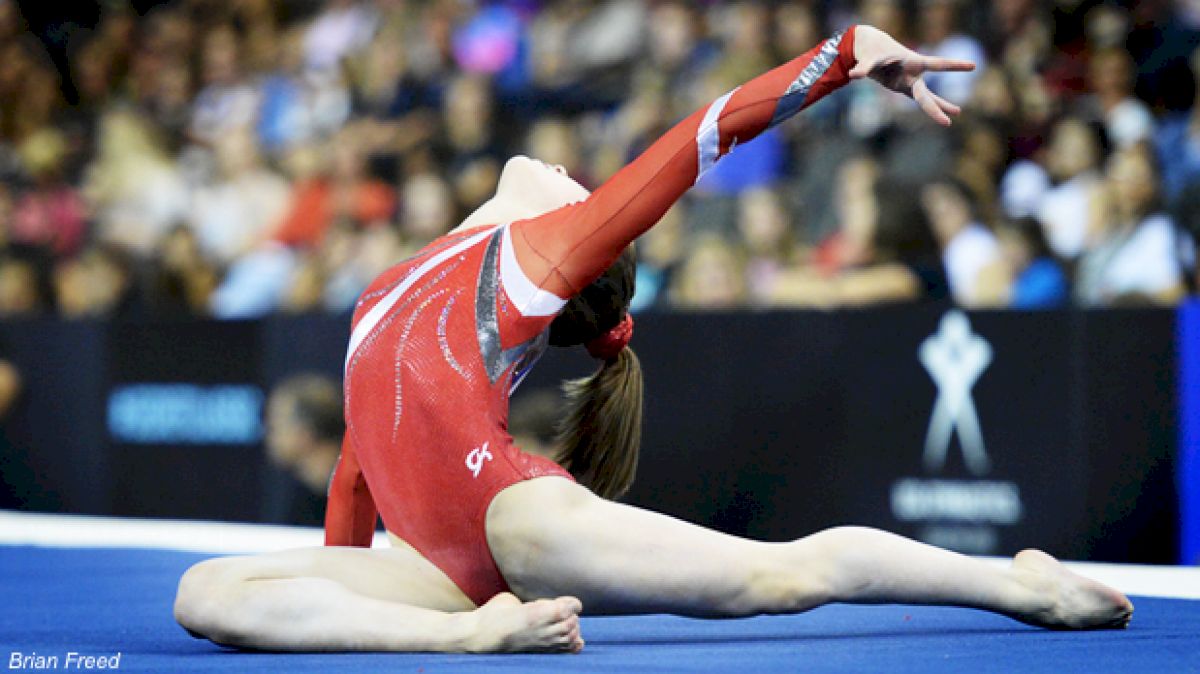The image captures a dynamic moment of a gymnast mid-routine on a blue mat. She is a young woman with long, brown hair tied up in a high ponytail using a red elastic. She wears a long-sleeved red leotard adorned with white, black, and silver accents, including a sheer red mesh on the sleeves and sparkly designs on the bodice. The gymnast is in a striking pose—her right leg is curled under her, foot pointed to the left, while her left leg extends straight back. Her back arches dramatically, and her head tilts back towards the floor, as she props herself up with her right arm and stretches her left arm high into the air, her hand flexed. The background is out of focus but densely populated, suggesting she is performing in front of a large audience. The image is credited to Brian Freed, noted in small white text at the bottom left corner.